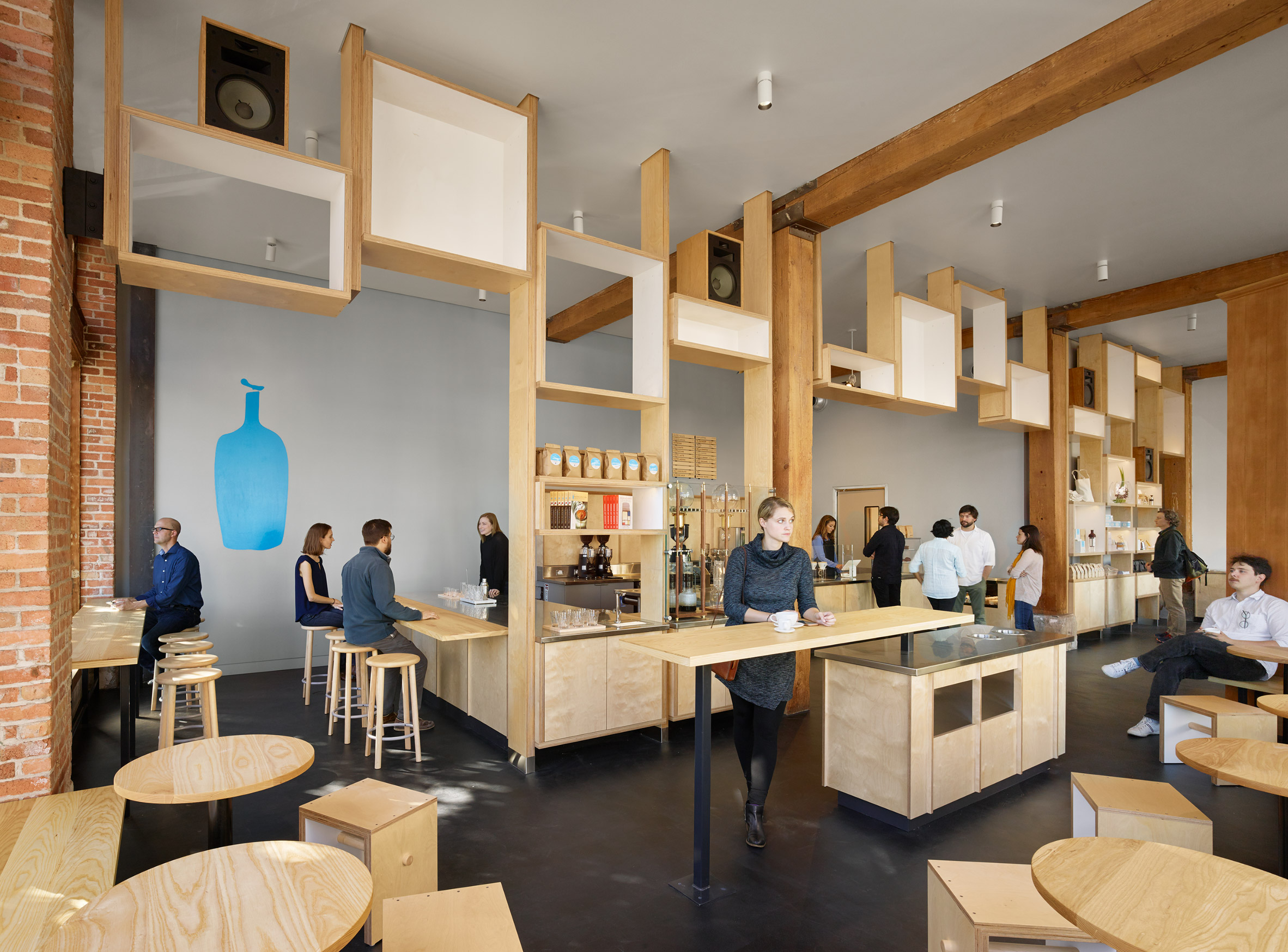The image depicts the interior of a modern, trendy coffee shop characterized by its spaciousness and minimalist decor. The coffee shop features tall white ceilings and a mix of white and exposed brick walls. Among the decor, a prominent blue art piece resembling a bottle is mounted on the wall. The flooring is a sleek, dark gray or black, which contrasts with the light-colored wooden furniture scattered throughout the space.

In the foreground, a young woman dressed in a gray long-sleeve sweater dress with boots stands with her brown purse and a white coffee cup on a wooden table. She seems to be interacting with the environment rather than sitting. Nearby, several young adults are seated on wooden stools and benches, some placed near large windows and others along bar counters. One man, casually dressed in a white polo shirt, jeans, and white tennis shoes, leans against the wall with a relaxed demeanor, holding a white coffee cup.

Towards the back of the cafe, a barista clad in a black apron over a blue long-sleeved shirt is stationed behind the counter, attending to customers. Coffee machines and bags of coffee are visible behind her, reinforcing the establishment's focus on beverages. Another barista, also dressed in black, is engaging with customers. The ambiance is lively, with groups of people chatting and waiting in line, while others peruse items displayed on shelves, which likely include coffee accessories and books. 

This detailed snapshot exudes the essence of a bustling yet inviting coffeehouse frequented by a young, vibrant crowd.